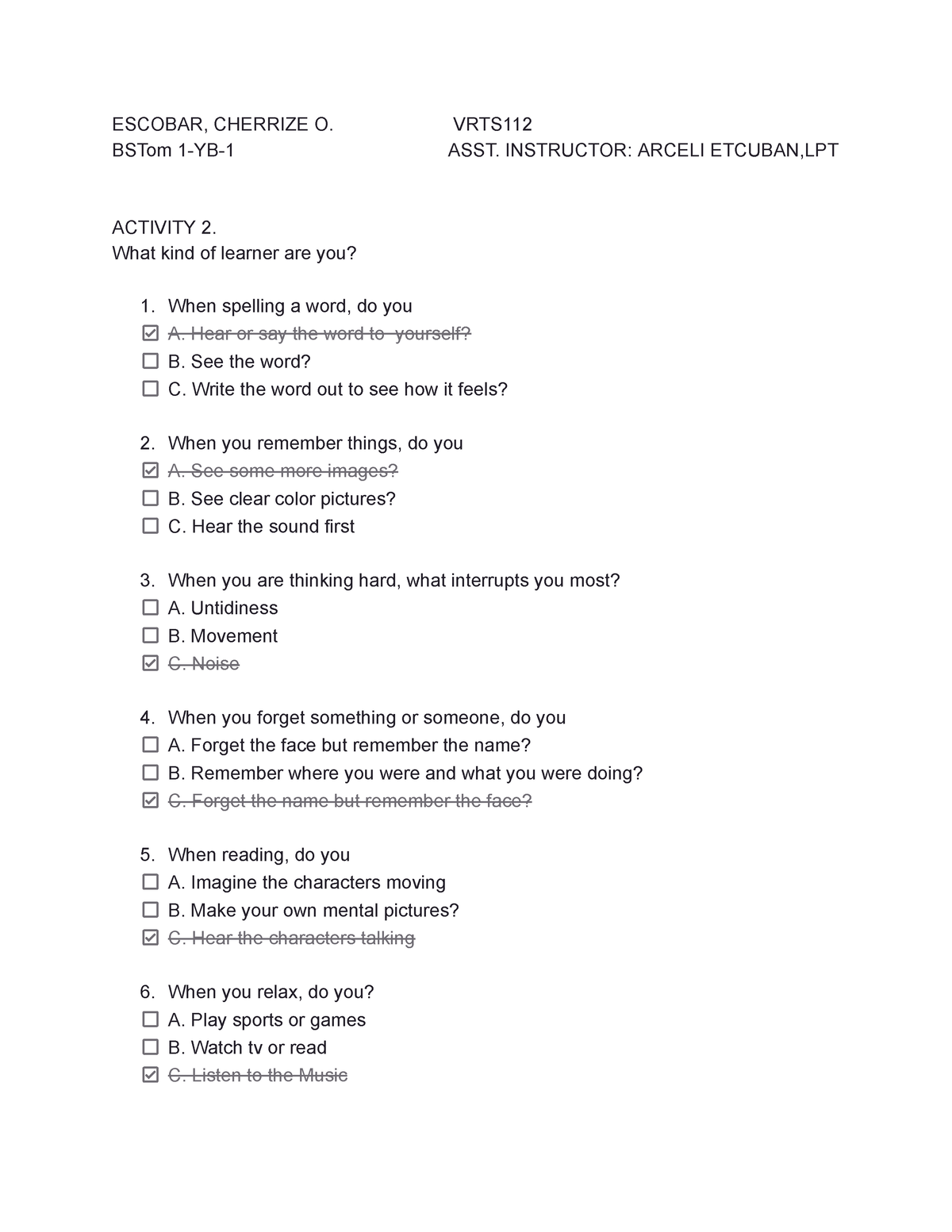**Caption:**

The document appears to be an educational assessment form, likely intended for students to determine their learning styles through a series of multiple-choice questions. At the top, spaces for the student's last name and first name are filled in with "Escobar, Cherise," suggesting the student might be Hispanic. The document includes several reference codes such as "VSTOM 1YB1" and "VRTS112." The assistant instructor listed is Ursula E. Tukubin, identified with the credentials "LPT."

The form, labeled "Activity Two," is titled "What Kind of Learner Are You?" and includes a series of six multiple-choice questions:

1. When spelling a word, do you:
   - A. Hear or say the word to yourself (this option is checked with a line through it)
   - B. See the word
   - C. Write the word out to see how it feels

2. When you remember things, do you:
   - A. See some images (checked)
   - B. (option not detailed)
   - C. (option not detailed)

3. When you’re working hard, what interrupts you the most:
   - A. Untidiness
   - B. Movement
   - C. Noise (this option is checked with a line through it)

4. When you forget something or someone, do you:
   - A. Forget the face, but remember the name
   - B. Remember where you are and what you were doing
   - C. Forget the name, but remember the face (this option is checked with a line through it)

5. When reading, do you:
   - A. Imagine the characters moving
   - B. Make your own mental pictures
   - C. Hear the characters talking (this option is checked with a line through it)

6. When you relax, do you:
   - A. Play sports or games
   - B. Watch TV or read (option not detailed)
   - C. Listen to music (this option is chosen)

The document is printed with black text on a white background, typical of a test or assessment form.